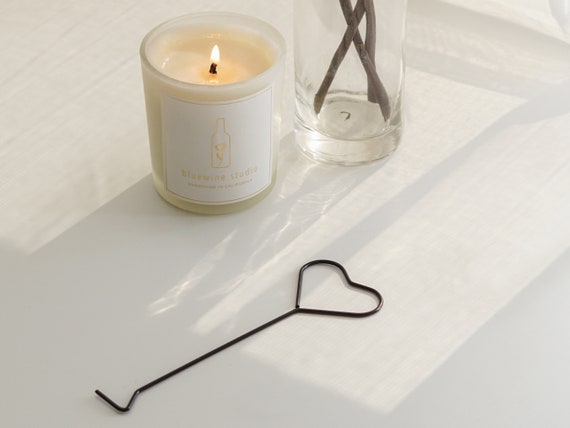The image depicts a serene still life on a white table, illuminated by sunlight streaming through a nearby window. On the upper right, a partially visible glass vase filled with brown stems casts soft gray shadows. Adjacent to the vase, a cream-colored candle with a lit wick and a yellow flame adds a warm glow. The candle's label features an image and text, though indistinct. Below these items, a black metal wire forms a heart shape and extends into a hook at the lower left. The overall scene is characterized by minimal color—white surfaces, gray shadows, cream from the candle, brown stems, and black wire—creating a cozy and tranquil atmosphere.